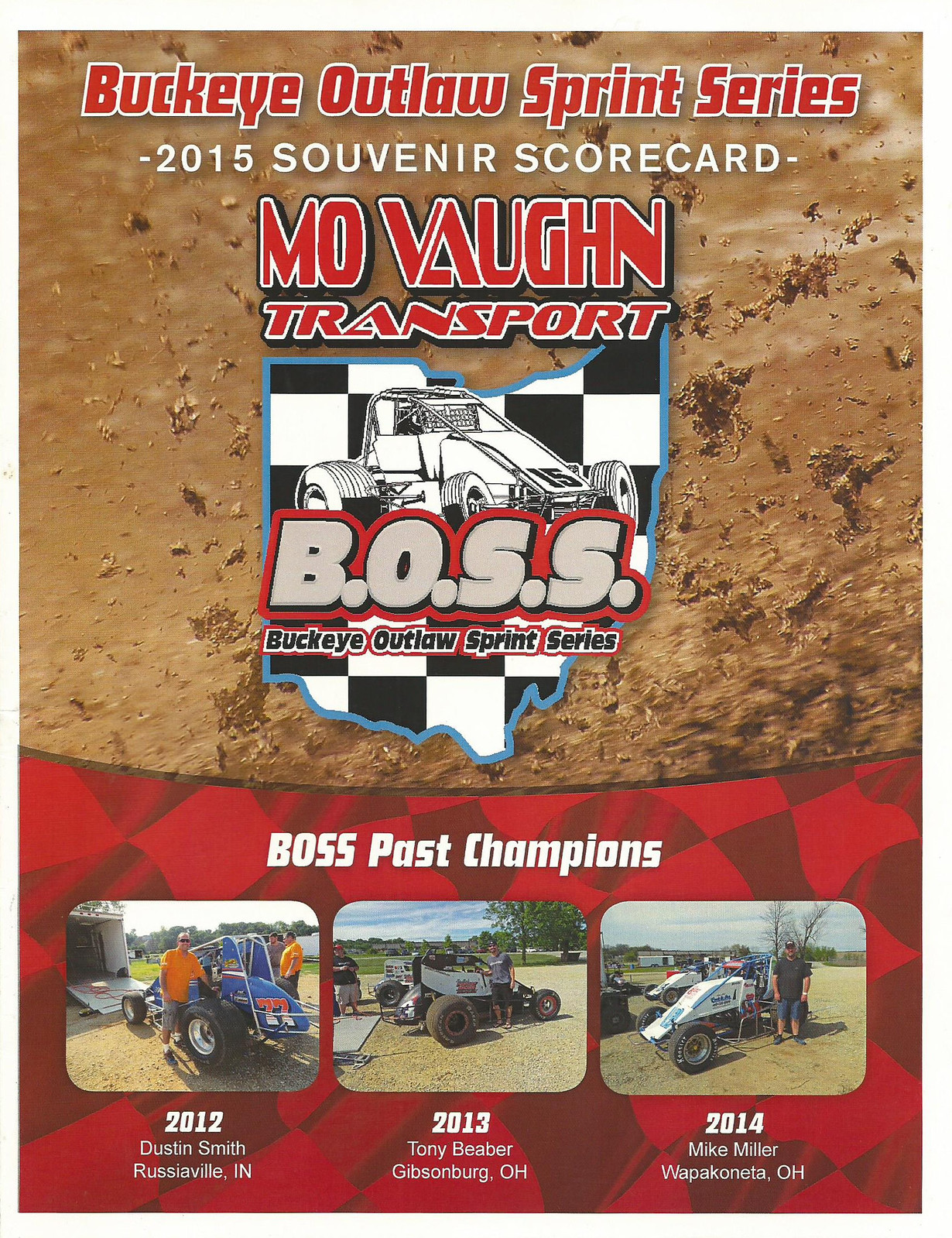The poster appears to be an advertisement or informational piece for the Buckeye Outlaw Sprint Series, specifically featuring a 2015 Souvenir Scorecard. The top portion has a brown muddy splash backdrop with bold red letters outlined in white that read "Buckeye Outlaw Sprint Series." Below this, "2015 Souvenir Scorecard" is written in white. Centered on the same muddy background, in red letters bordered in white, it reads "Move On Transport." There is an artistic rendering of a racing buggy, set within an outline of the state of Ohio, which has a checkered interior. The initials "B.O.S.S." stand prominently, representing the Buckeye Outlaw Sprint Series.

The lower portion of the poster transitions into a red checkered flag background. Here, in white text against red, it reads "BOSS Past Champions." This section features three pictures of men standing beside their racing buggies. Each photo marks a different year and the respective champion: "2012, Dustin Smith, Rushaville, Indiana," "2013, Tony Baber, Gibsonburg, Ohio," and "2014, Mike Miller, Waukeconeta, Ohio."